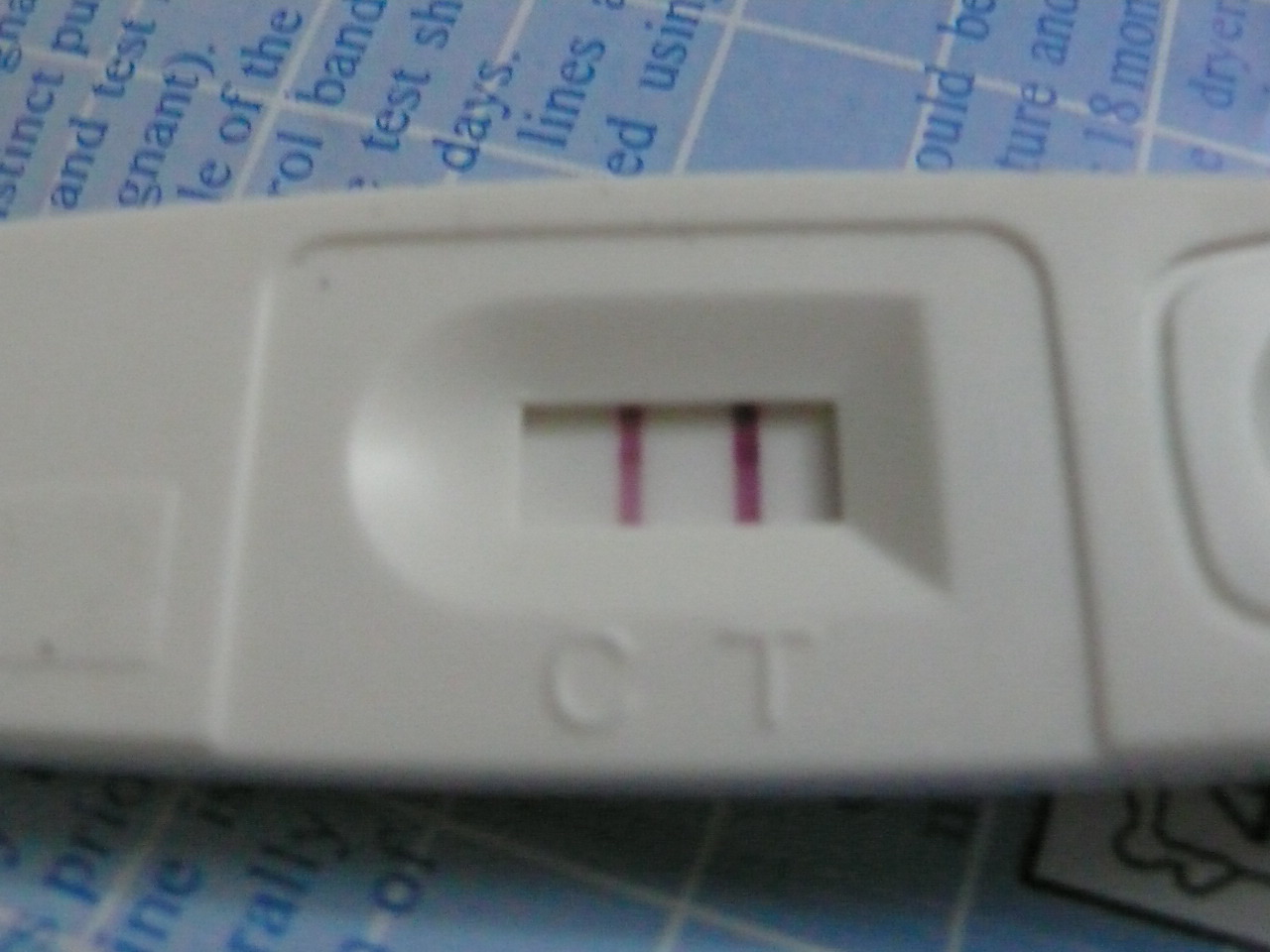A close-up photograph captures a pregnancy test made of thick white plastic. The test displays the imprinted letters "C" and "T" at its base, surrounding a small indicator window above. Within this window, two medium-thickness lines appear in a deep, crimson red with a faint purplish hue. The line on the left is slightly fainter than the one on the right, but both remain bold and easy to discern. Due to the zoomed-in nature of the image, the test itself is slightly out of focus, introducing a minor blur that contrasts with the clearer background. The test is placed atop a pamphlet or booklet, featuring blue text mostly obscured by the test. Visible words such as "pregnant," "test," and "days" suggest the pamphlet provides instructions. The pamphlet's surface is adorned with a subtle light gray and blue grid pattern, intersected by white lines.